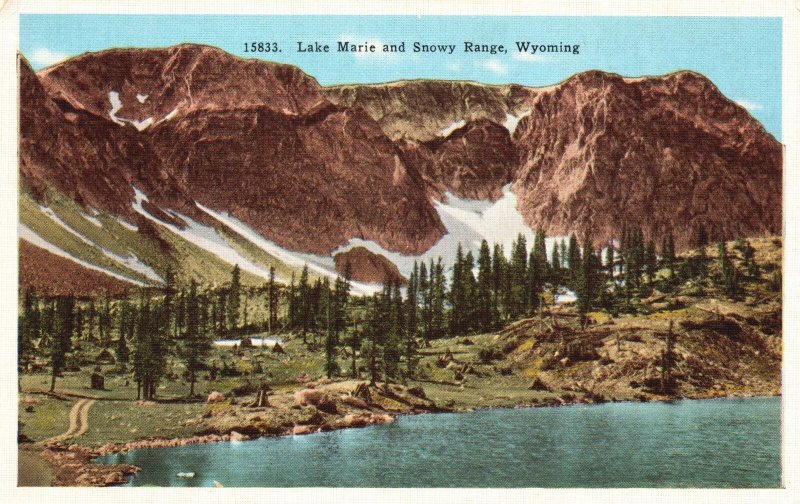This horizontal, vintage postcard-style print titled "15833. Lake Marie and Snowy Range, Wyoming" captures a breathtaking natural scene in exquisite detail. A thin beige border frames the image, enhancing its classic aesthetic. 

In the foreground, a calm, teal-colored Lake Marie barely ripples, reflecting its serene surroundings. Flanking the lake, a rocky shoreline transitions into a green grassy bank. As your eyes move up, a dirt hill dotted with tall evergreen trees forms a natural divide. The trees rise majestically, creating a lush green line just before the rugged mountain backdrop.

Dominating the scene is the Snowy Range, a dramatic mountain landscape characterized by earthy, reddish-brown rocky peaks. These peaks are intermittently streaked with patches of snow, nestling in the crevices and valleys between them. The mountain's rugged terrain appears both imposing and beautifully wild. Above, the sky is a crisp blue, dotted occasionally with wisps of white clouds, completing this picturesque Wyoming tableau.

This meticulously detailed image not only captures Lake Marie's tranquil beauty but also the imposing grandeur of the Snowy Range, creating a vivid and immersive glimpse into this stunning natural setting.